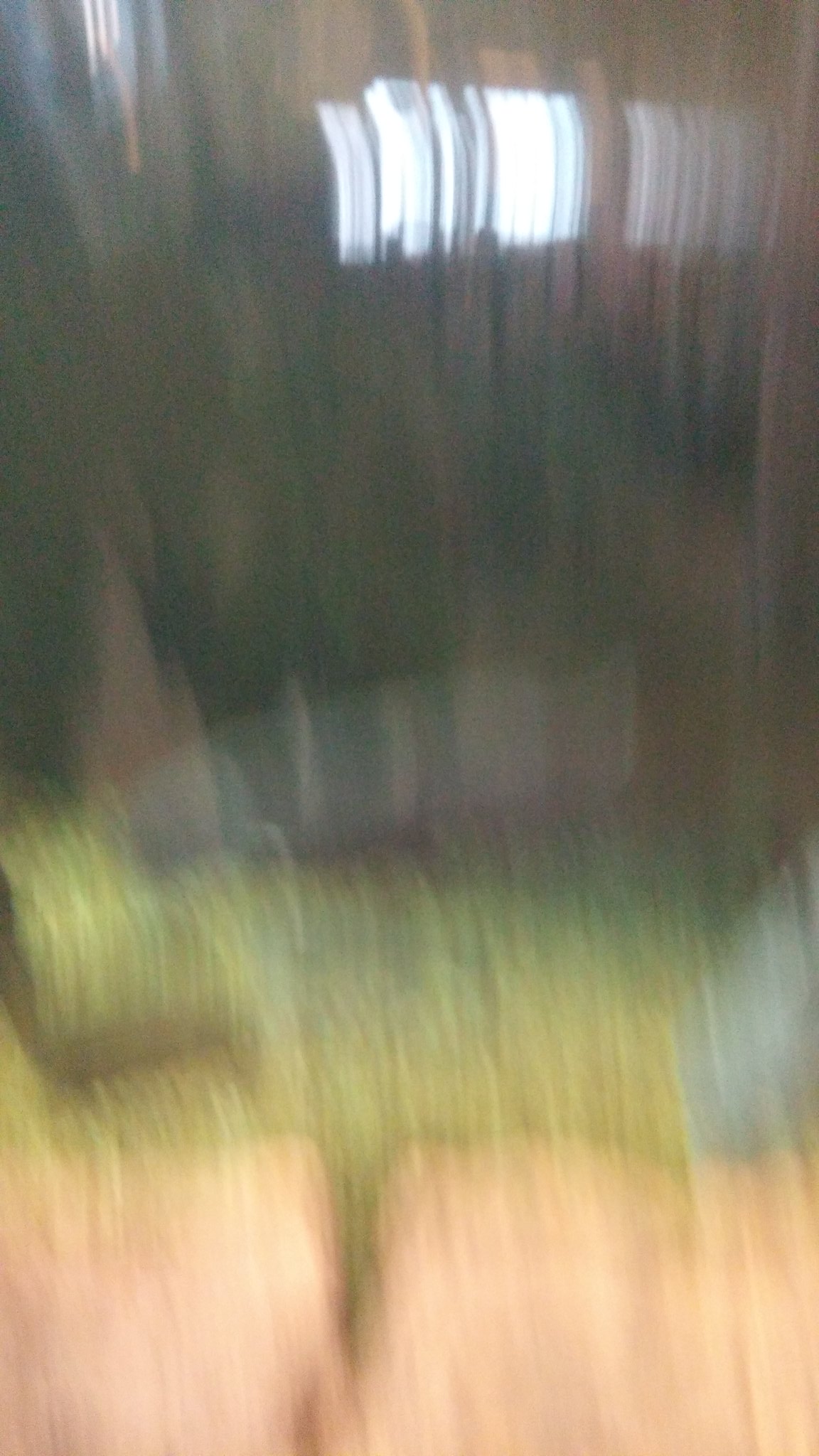This photograph, taken close to or during the evening, presents a mosaic of blurred colors and shapes, likely due to movement when the picture was snapped. The scene appears to be outdoors, showing a person moving along a sidewalk composed of concrete pavers with distinct separations. The pavers look light gray or light brown under uneven lighting. To the right, there's a patch of grass showcasing varying shades of green, intermingled with a bluish-gray object. 

The image's blurriness intensifies towards the edges, particularly on the left, with smears of dark green, light gray, dark gray, light brown, and red. In the upper portion of the photograph, blurred dark shapes suggest a possible window with a cyan blue tint fading to white, partially obscured by a thin, curtain-like object. Beneath the window, the movement creates a ghostly impression of flesh-colored forms, resembling someone's fists, transitioning into a light tannish-green area with some gray. Darker elements at the top hint at interior items such as windowsills and possibly a person or objects near a window, but everything remains indistinct and lost in the blur of motion.